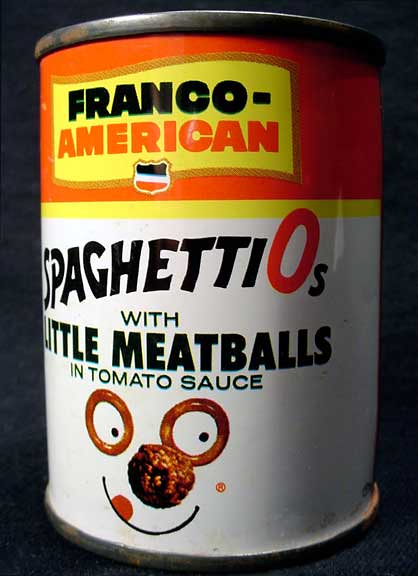This image showcases a vintage can of SpaghettiOs by Franco-American. The top portion of the can features an orange band with a yellow flag emblazoned with "Franco" in black and "American" in orange lettering. Beneath this, a yellow line separates the orange top from a white background below. Prominently displayed in black font is the brand name "SpaghettiOs," with the "O" designed in eye-catching orange, mimicking the pasta shape. Below this, it reads "with little meatballs in tomato sauce" also in black lettering. The lower portion of the can boasts a playful face made from the product: two SpaghettiO noodles with black pupils serve as the eyes, a meatball forms the nose, and a small, semi-circle mouth with a pink dot acting as a tongue completes the face. The entire image is set against a black background, effectively highlighting the nostalgic can of SpaghettiOs with little meatballs.